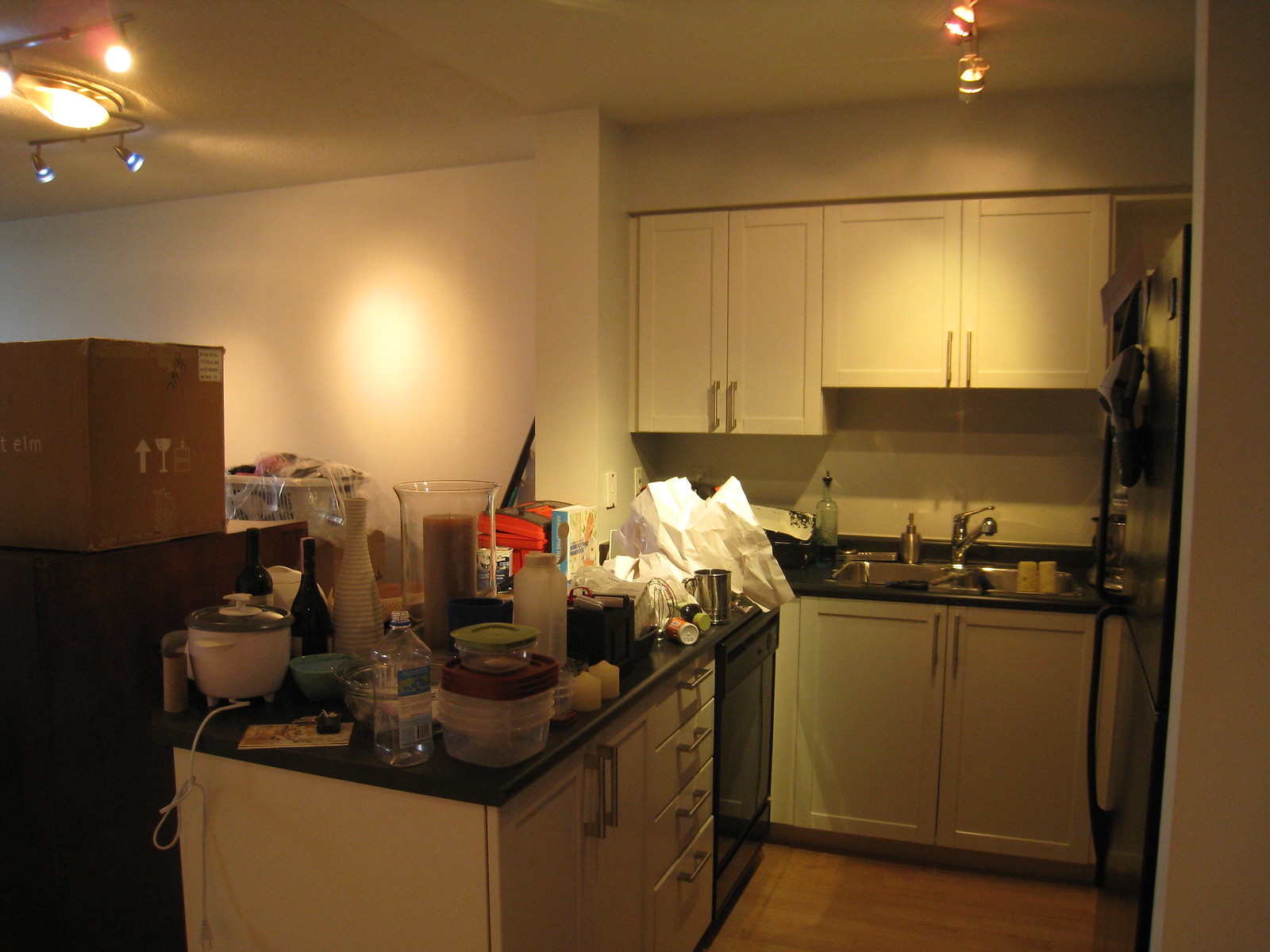In the image, a dimly lit kitchen and adjoining dining room are depicted, creating an intimate and somewhat cluttered atmosphere. The kitchen, predominantly decorated in white and cream hues with dark accents, features a central island and countertop heavily laden with an assortment of kitchen tools, bottles, canisters, packages, and cups of various colors and shapes. The back wall of the kitchen is lined with upper and lower cabinetry, and positioned between the cabinets is a sink with a faucet, where a bottle of dish liquid and a pile of unwashed dishes are visible. To the left, the furnishings blend light and dark brown tones, adding a warm contrast to the otherwise pale decor. Above, the lighting arrangement includes four spotlights centrally focused on the kitchen area, complemented by additional lights to the left that illuminate the walls. A large central spotlight is flanked by smaller spotlights, creating a multifaceted light scheme that, despite its presence, fails to significantly mitigate the overall dimness of the scene.